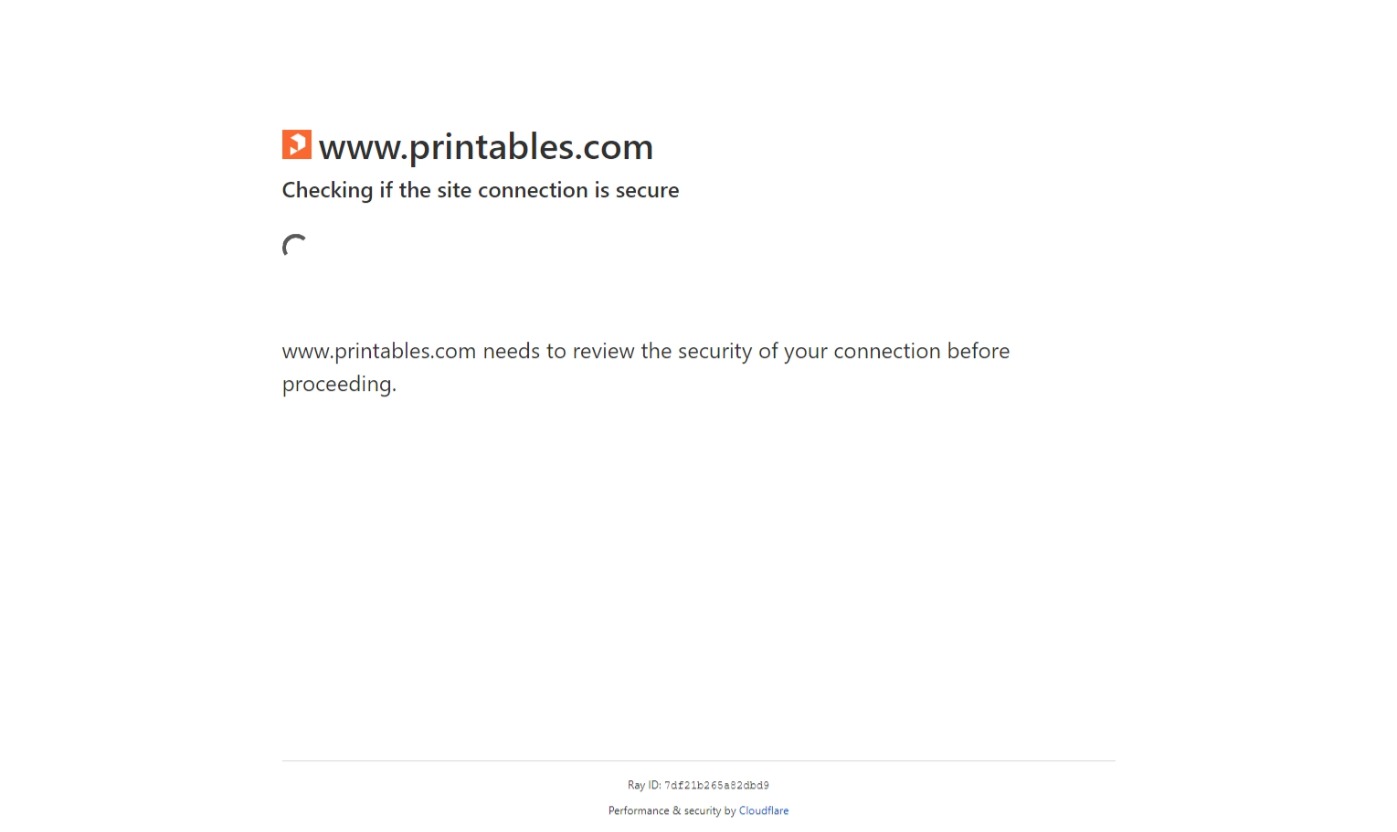The image depicts a notification screen or pop-up typical of a website, occupying a white background. In the top left corner, there's an orange square featuring a white icon. Immediately to the right, bold black text reads "www.printables.com."

Beneath this, aligned to the left, the text states, "Checking if the site connection is secure." Below this message, a blank white space dominates, except for a left-aligned black half-circle loading icon which appears to be in a spinning or loading animation.

At the bottom, the notification states, "www.printables.com needs to review the security of your connection before proceeding," followed by an identification note secured by Cloudflare.